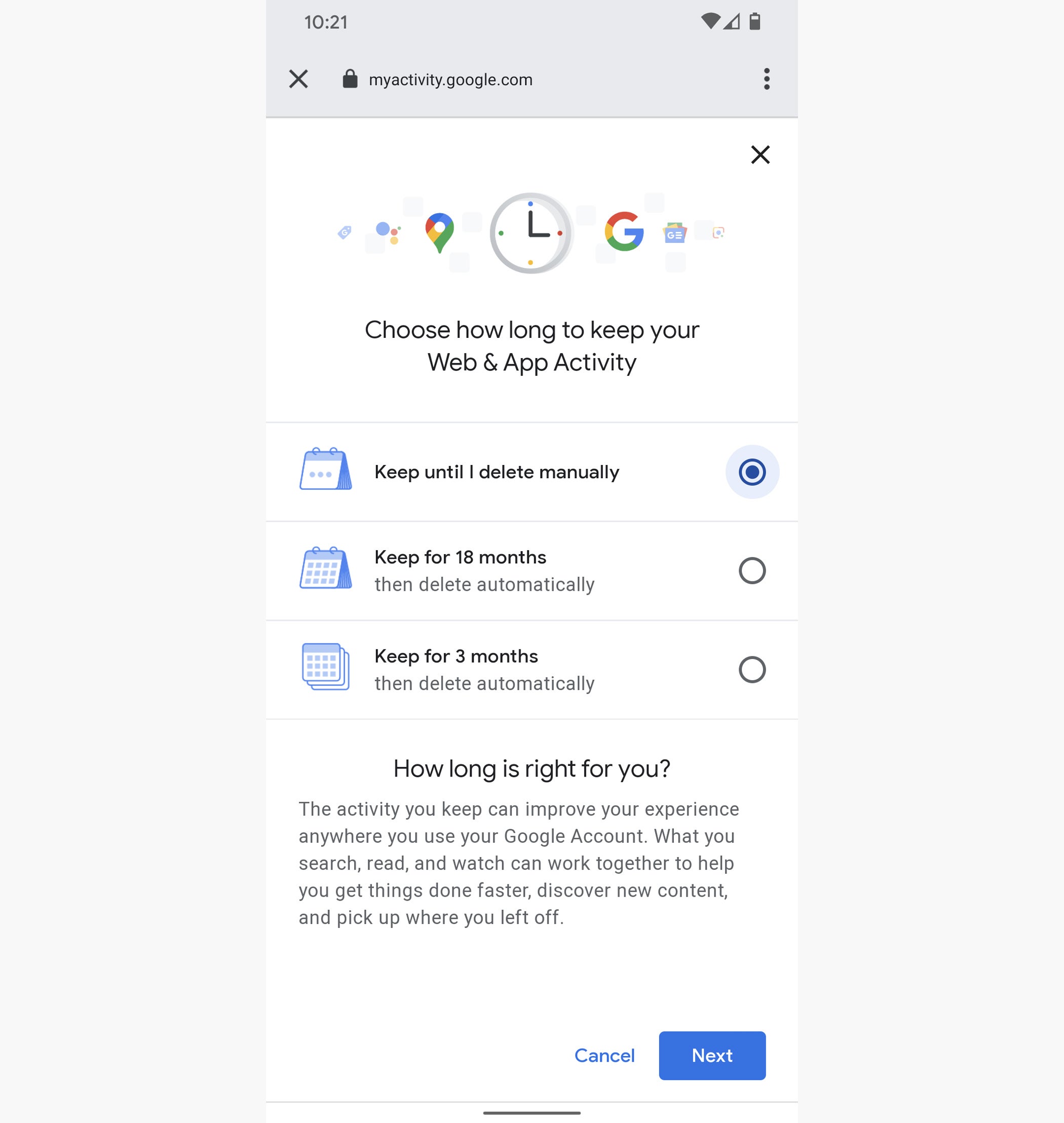The image displays a user's screen showing their Google activity settings. The top of the screen features icons indicating a Wi-Fi connection (though not at full strength) and a partially drained battery. An 'X' and a lock icon are also visible. The URL "myactivity.google.com" is displayed prominently alongside a stack of dots symbolizing a menu.

The main section of the screen is focused on the "Web & App Activity" settings. The user is presented with an option to "Choose how long to keep your web and app activity." Below this, various retention choices are shown. A blue checkmark indicates the current selection to "Keep until I delete manually." Other options include "Keep for 18 months" and "Delete automatically." The screen also mentions a calendar and a specific setting to keep activity for 3 months.

There is explanatory text highlighting that saving activity can enhance user experience by allowing Google services to offer more personalized suggestions and faster access to frequently used features. At the bottom of the screen, buttons for "Cancel" and "Next" are visible.